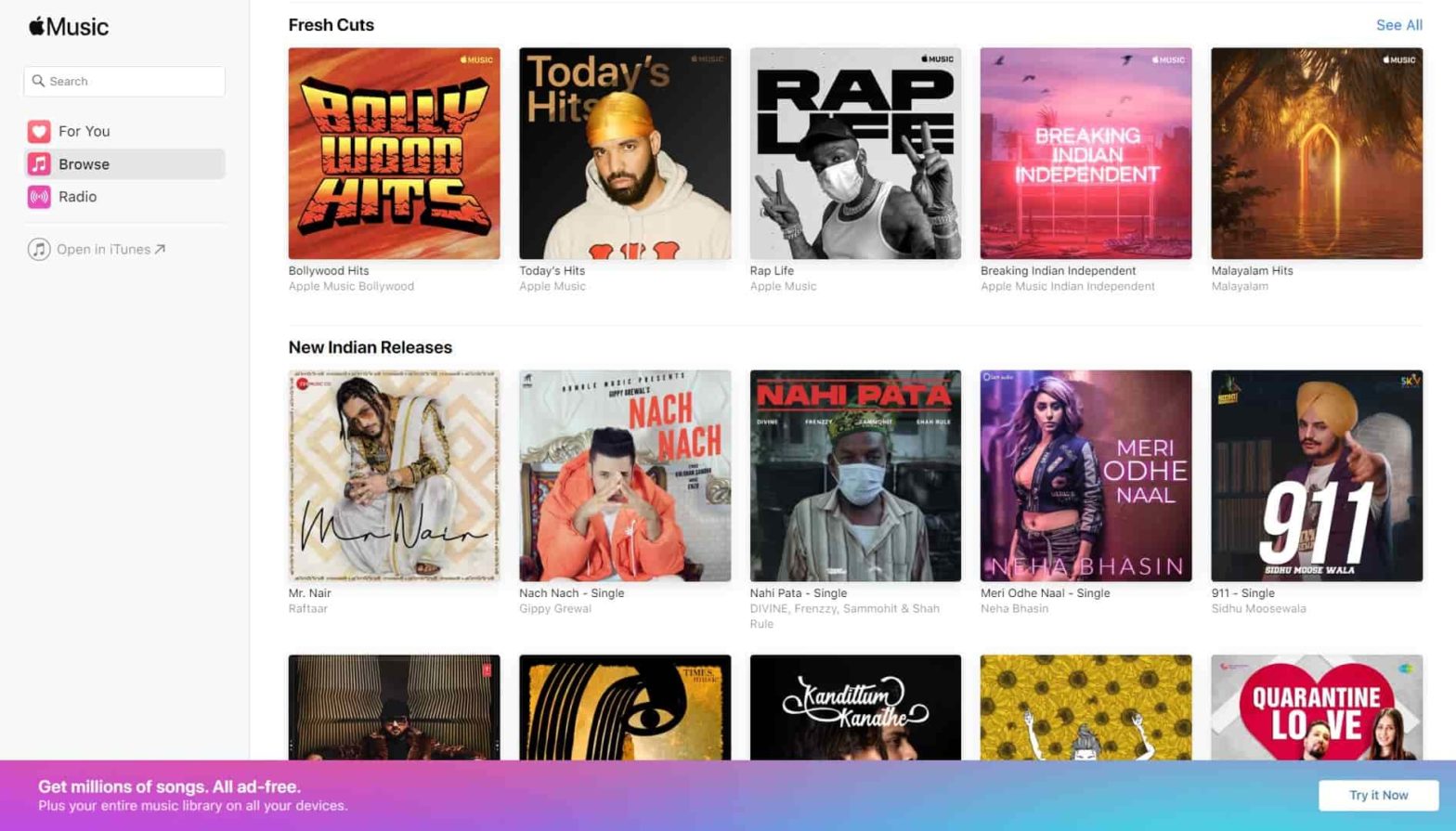The image displays an Apple Music interface, identifiable by the Apple logo and the word "Music" located in the top left corner. Adjacent to the logo, there is a search bar followed by three main navigation options: "For You" with a heart icon, "Browse" with a musical note icon, and "Radio." Beneath these, there is a clickable text option to open the app in iTunes.

The main content area features 15 album covers organized in three rows. The first row, titled "Fresh Cuts," showcases five albums with a "See All" option on the far right to view more albums in this category. The second row highlights a selection of Indian releases, again displaying five albums. The third row includes an additional five albums, although the entire images of the albums are not fully visible.

At the bottom of the screen, a banner prominently advertises "Get Millions of Songs All Ad-Free" with a "Try It Now" button situated on the far right. The albums predominantly feature Indian music artists, indicating a diverse musical selection available on Apple Music.